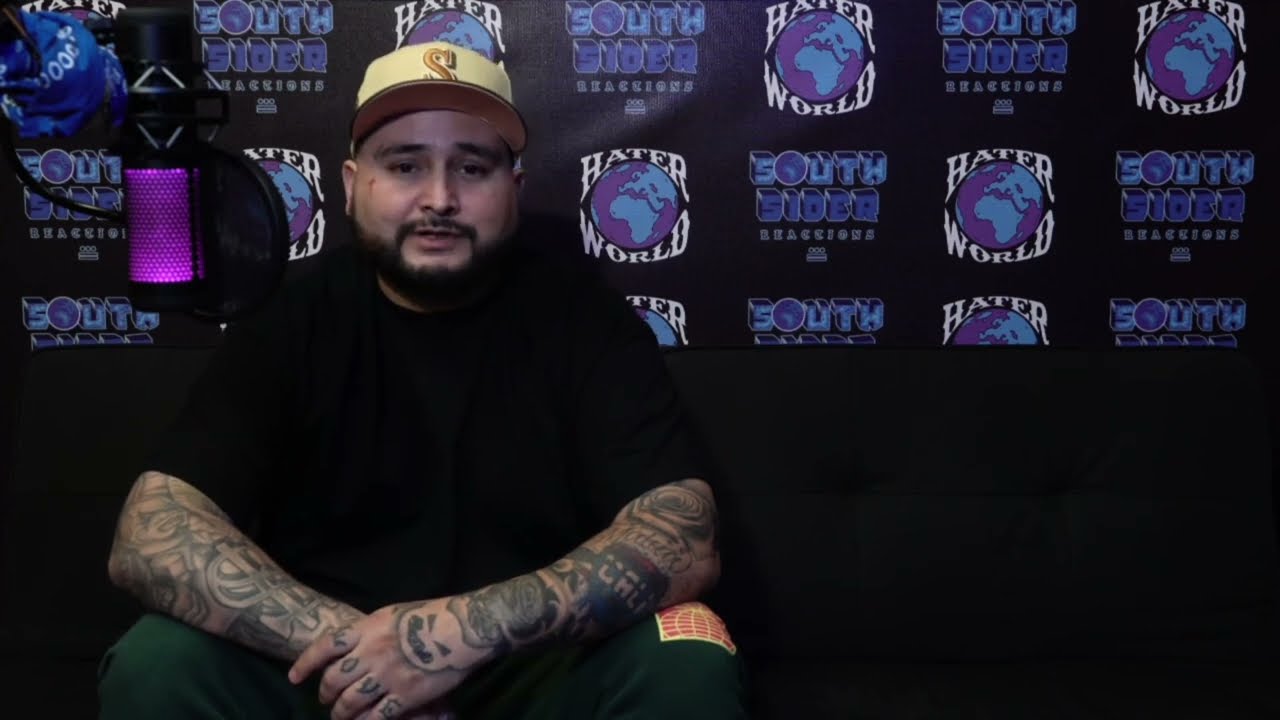A photograph features a man of Hispanic descent sitting down slightly to the left of center. He is facing the camera with his elbows resting on his thighs and his hands clasped together, left hand over the right. He sports a yellow baseball cap with a brown "S" on it, tilted slightly upwards, casting an orange-tinted shadow underneath the brim. His attire includes a black shirt and green pants, the latter adorned with a yellow patch speckled with light red spots. His brown skin is complemented by a full black beard and mustache, and his arms are covered in extensive tattoos, including letters on his fingers that spell out the word "love." In the background, against a predominantly black wall, there are advertisements featuring two brand names, "Hater World" and "Southside." "Hater World" is displayed in white text around an emblem of the Earth, while "Southside" features a blue gradient with an "O" represented by an Earth image. The advertisements are staggered and create a patterned backdrop. Additionally, there is a bright purple illuminated cylinder off to the left behind the man. The photograph is widescreen, resembling the dimensions of a high-definition TV.